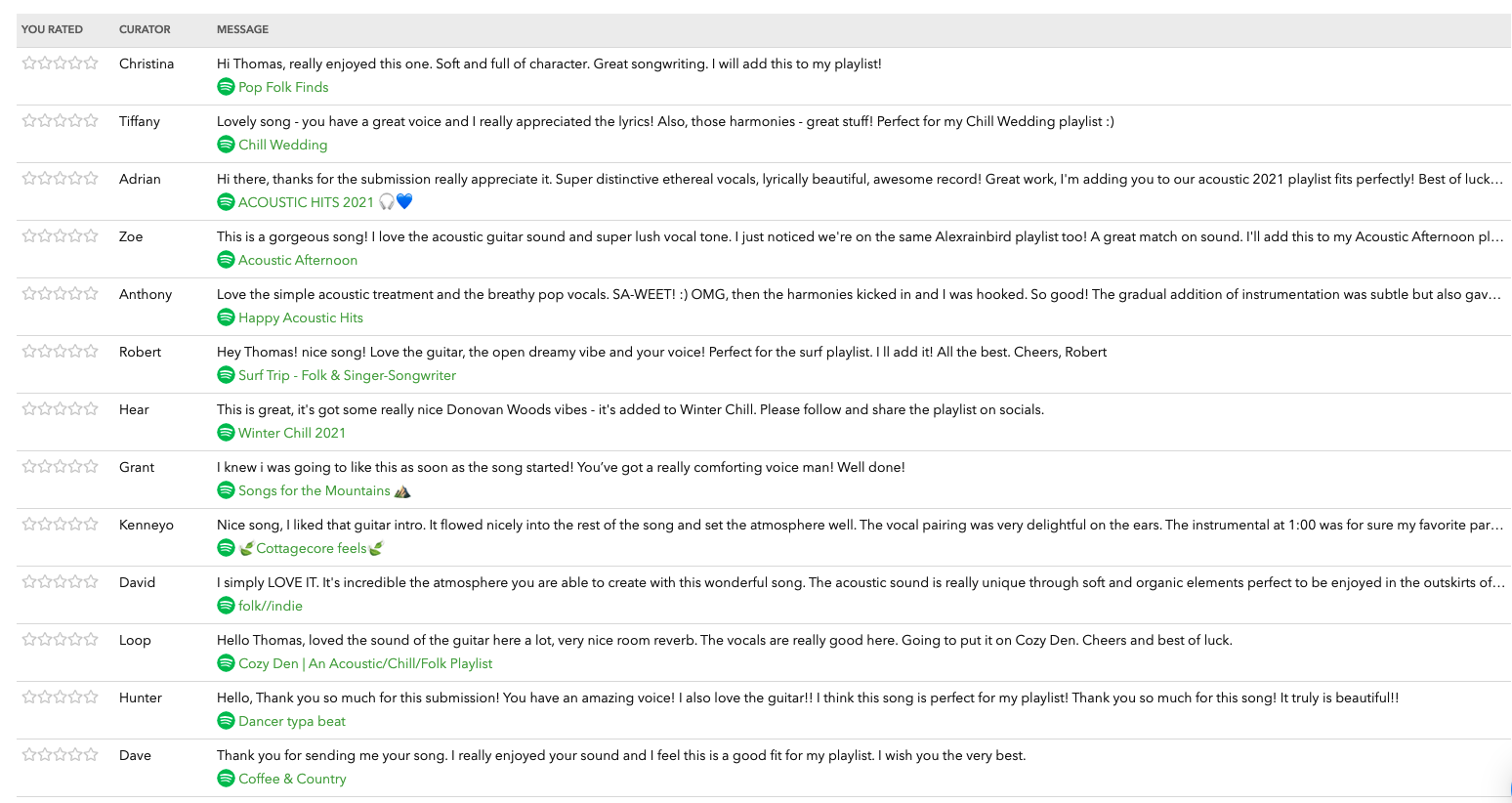The image depicts a messaging interface displayed on a white background. At the very top, there's a duration indicator, while directly below it, a partially obscured word appears due to a prominent save icon with a pin symbol above it. 

Following this, a grey bar spans across the top of the interface labeled "Message." Beneath the grey bar, several messages are listed in black text. For each message, the subject line is highlighted in green with a small circle next to it. 

An example of a message reads: 
- "Hi Thomas, really enjoyed this one. Soft and full of character. Great songwriting. I will add this to my playlist," followed by the subject "Pop Folk Finds."

To the left of each message, the sender's name is displayed. Adjacent to the names are five stars, which appear unhighlighted, suggesting an option to rate the messages by clicking on the stars. 

In total, there are 13 messages from different individuals, including Christina, Tiffany, Adrienne, Zoe, Anthony, Robert, Here, Grant, Kenny O, David, Luke, Hunter, and Dave. The interface's sole color accents are the green highlights used for the subject lines of the messages.